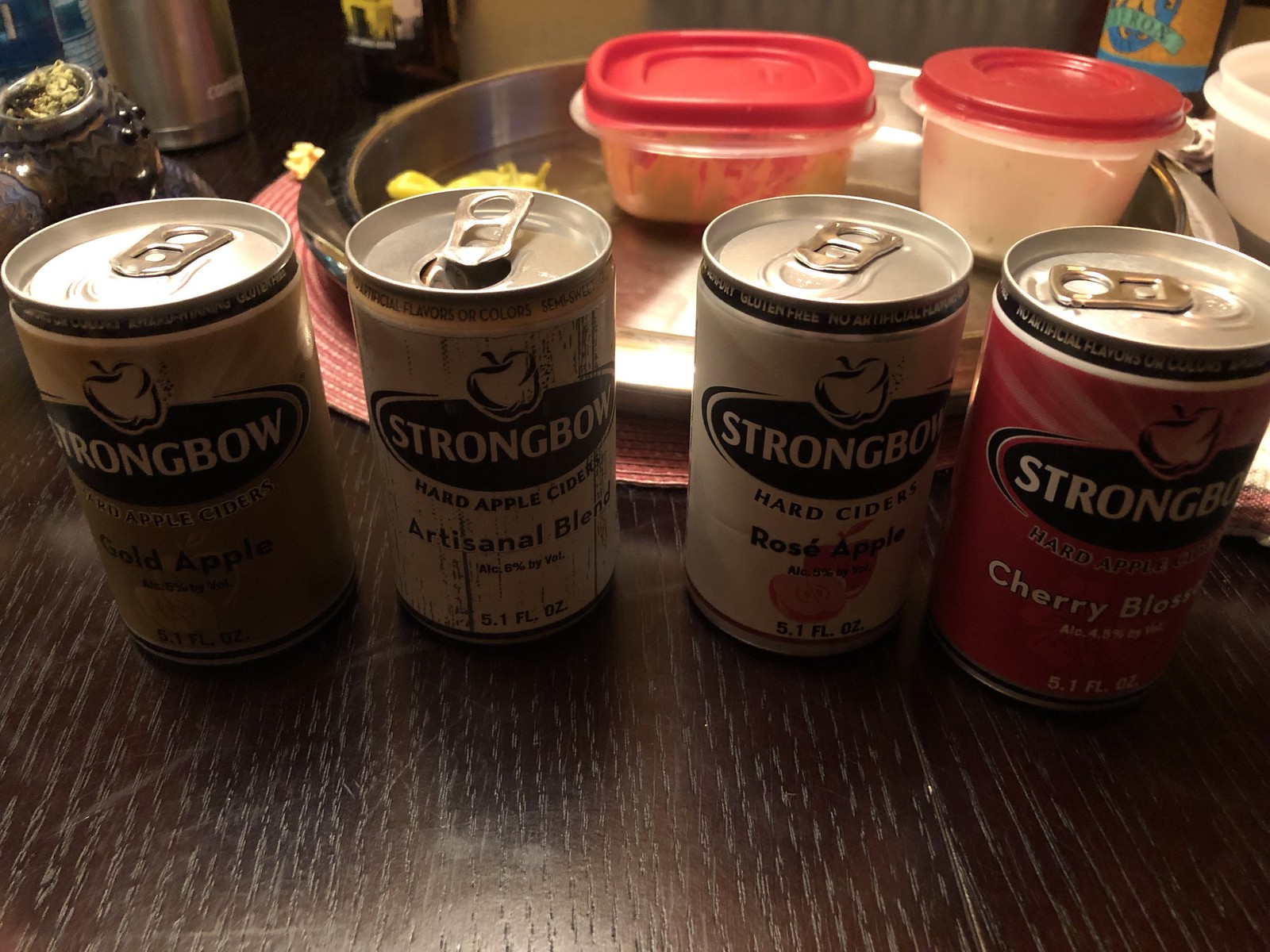The image depicts a residential kitchen workspace featuring a tabletop with four cans of Strongbow hard cider arranged in a line, their labels facing the viewer. The cans—one open and three closed—showcase various flavors, including a cherry blend and an artisanal blend. The three cans on the left have brown labels, and the one on the right has a dark red label. Behind the cans, there is a large silver pan holding a round black serving tray. On the tray are two Tupperware containers with red lids, a square one and a bowl. The kitchen background includes a reflective surface and possibly a pipe in the upper left corner. To the far left of the image, a ceramic figure can be seen, adding to the residential feel of the setting. The backlighting makes some of the details less legible, contributing to a slightly mysterious atmosphere.